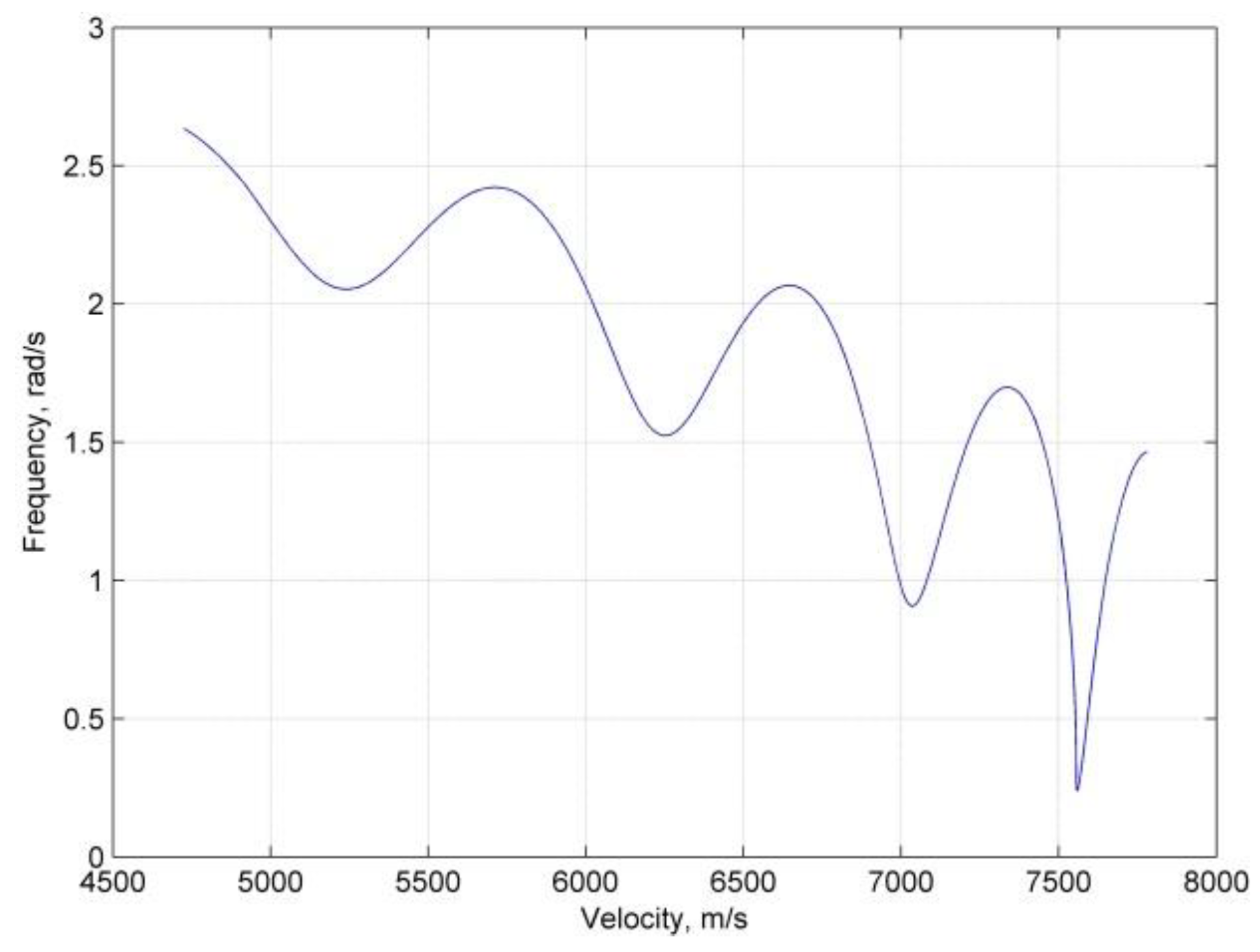The image displays a detailed line graph against a grid background. The x-axis represents velocity in meters per second (m/s), ranging from 4,500 to 8,000 in increments of 500 (i.e., 4,500, 5,000, 5,500, and so on up to 8,000). The y-axis denotes frequency in radians per second (rad/s), ranging from 0 to 3 in increments of 0.5 (0, 0.5, 1, 1.5, 2, 2.5, 3). The graphed line, potentially blue or black, originates from the upper left of the graph at approximately 4,600 m/s and a frequency of 2.6 rad/s. The line exhibits multiple peaks and troughs as it progresses, reaching its lowest point at about 7,600 m/s and 0.2 rad/s. This marked dip is followed by a sharp rise, concluding around 7,700 m/s and 1.4 rad/s. The graph's numerous undulations depict a fluctuating relationship between velocity and frequency.